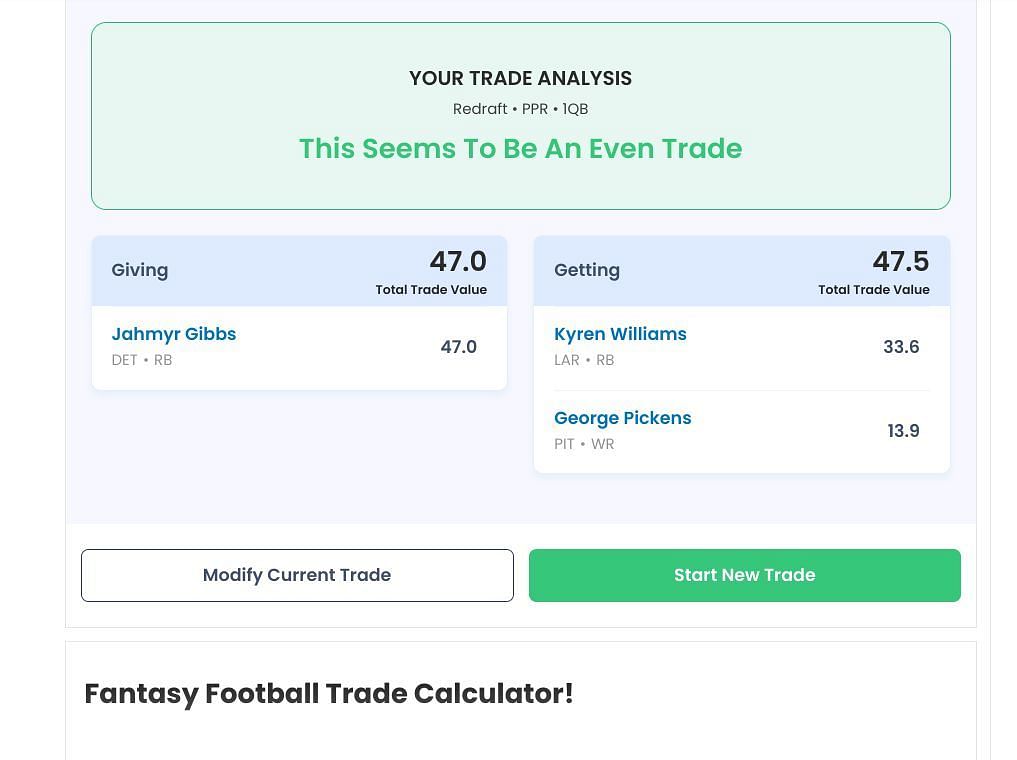The image appears to be a screenshot from an app or website, with dimensions that are roughly square. The top two-thirds feature a light blue background, while the bottom third shifts to white. 

Taking up approximately 25% of the image's height and spanning its full width, a rounded-rectangle with dark green edges transitions to a lighter green within. This rectangular section contains three lines of centered text. The first line, in black capital letters, reads: "YOUR TRADE ANALYSIS." The second line, in smaller, non-capitalized black text, reads: "Redraft • PPR • 1QB." The third line, in medium green text and larger font, proclaims: "This seems to be an even trade."

Below this rounded-rectangle, about one-third of the way down the image, there is another box on the left taking up roughly half the image’s width. This box has a slightly darker blue background and is divided into two sections. On the left, it reads "Giving," and on the right, it shows "47.0." Below this number, in smaller text, is the label "Total Trade Value."